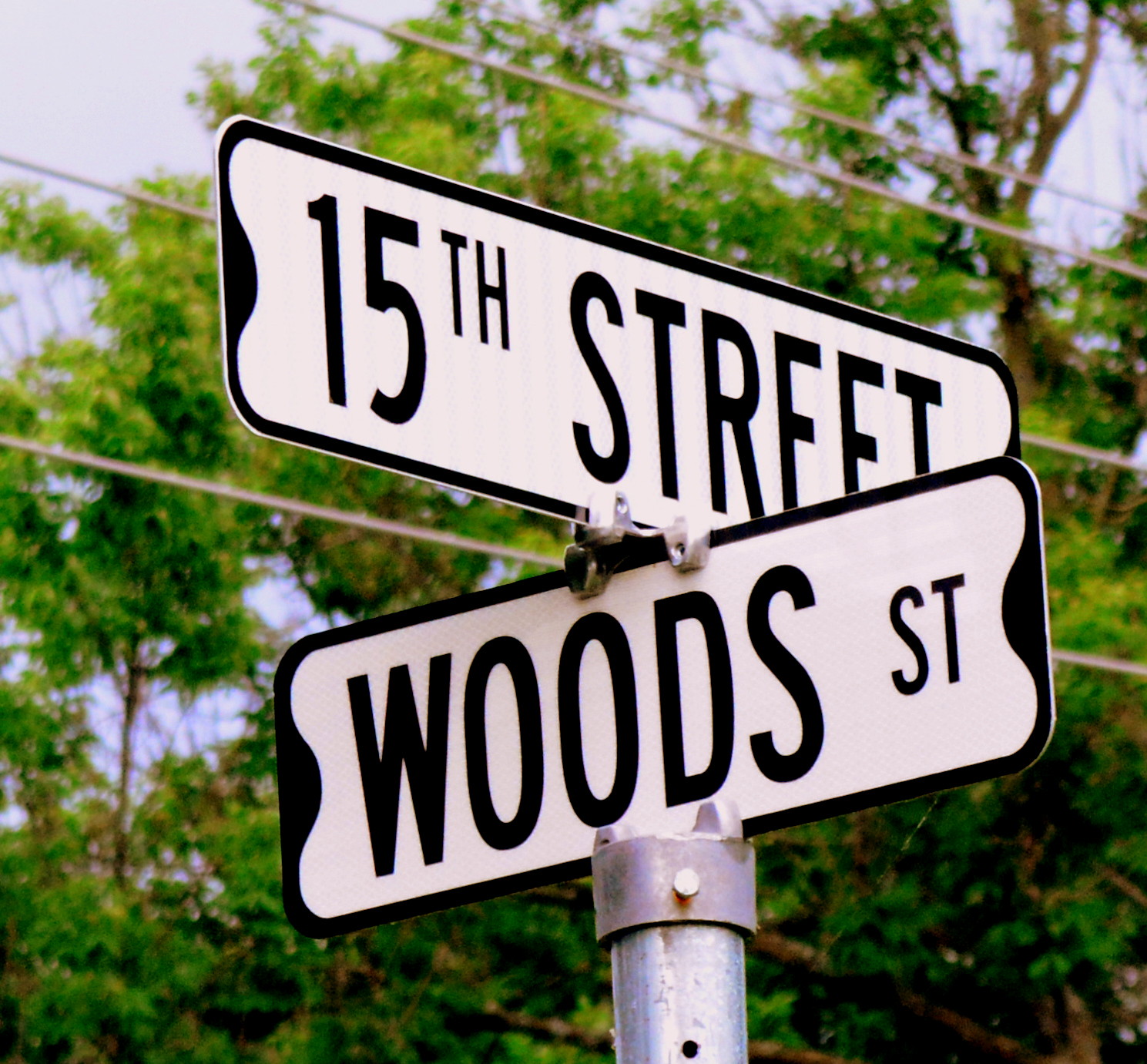A detailed description for the given image could be:

"This photograph prominently features a pair of intersecting street signs mounted on a metal pole. The top sign, which is horizontal and in black and white, displays '15th Street' in bold black lettering. Perpendicularly intersecting it is another black street sign for 'Wood Street.' The scene is set against a backdrop of intertwining power lines overhead, suggesting a network of electrical or utility lines. Behind the pole, towering trees with an abundance of green foliage provide a natural canopy, their bark visible on the lower section of the image. The vivid blue sky serves as a striking contrast to both the urban and natural elements in the photograph, emphasizing the clear, sunny weather."